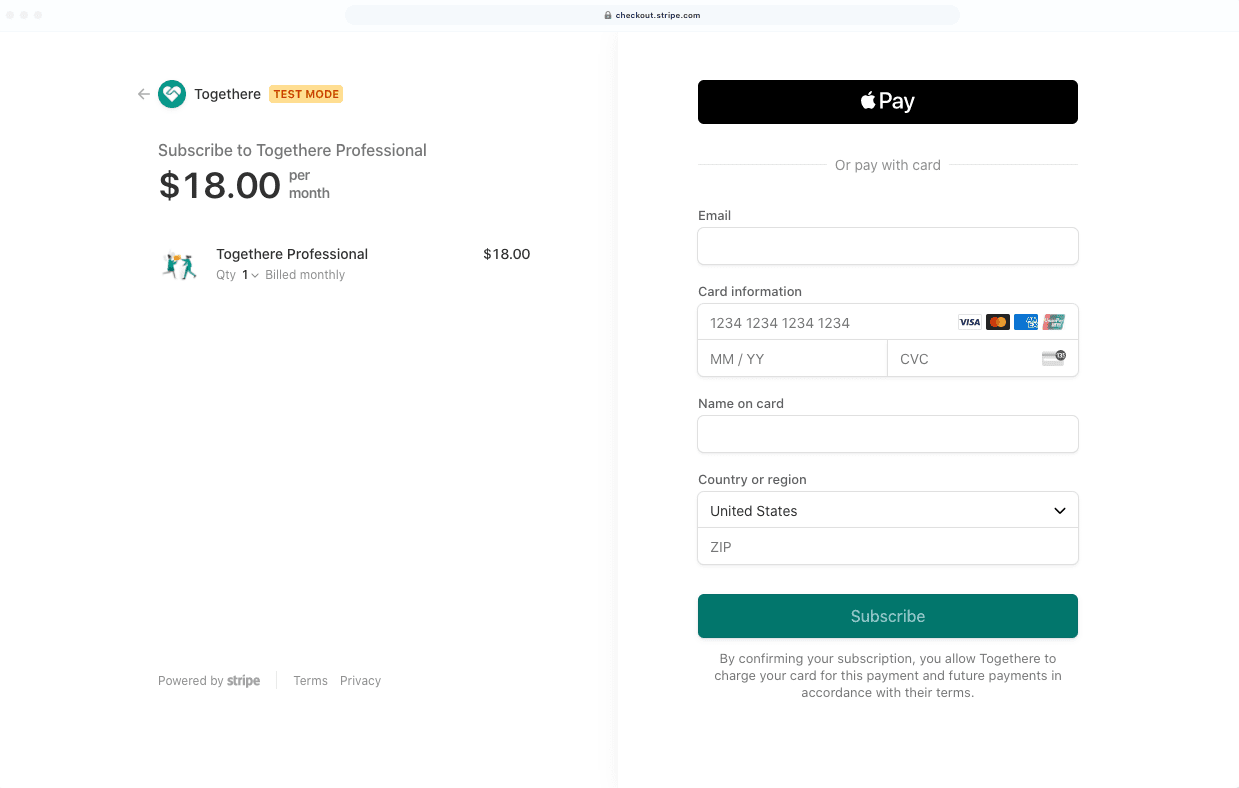The image shows an invoice that appears small and difficult to read. At the top of the invoice, the heading says "Together Ear," spelled as T-O-G-E-T-H-E-R-E. Beside this heading is a teal circle with a white heart inside it, and to the left, there's an arrow pointing left.

Below the heading, there's an orange rectangle with red capital letters that read "TEST MODE." Above this rectangle, there is a blue hyperlink that says "Check out stripe.com." Beneath the "TEST MODE" label, the text reads: "Subscribe to Together Ear Professional - $18 per month." Following this, it reiterates "Together Ear Professional - $21 billed monthly" and "$18."

To the right of this text, there's a black rectangle with a white Apple logo inside it, indicating the option to pay via Apple Pay. Additionally, there is text below stating "Pay with card," followed by fields labeled "Email" to enter an email address, "Card Information" to enter card details, and options to select the card type (Visa, MasterCard, American Express). Further fields are provided for the card's expiration date (month and year) and the CVC code.